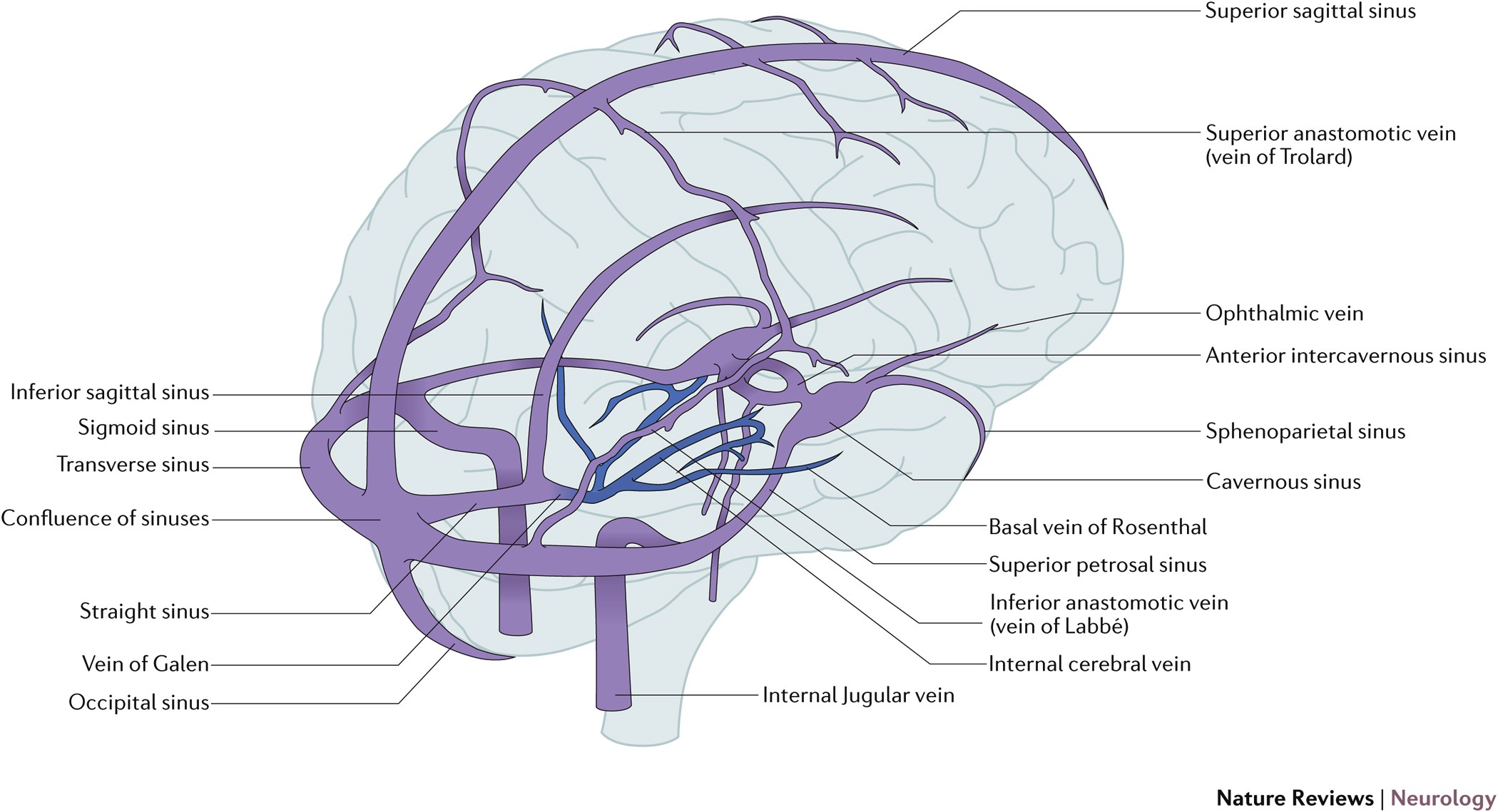This detailed diagram, likely from a medical textbook or educational chart, illustrates various veins in the human brain using shades of light, medium, and dark blue, with some veins depicted in a purplish-blue hue. The brain itself is colored in a grayish-blue, contrasting with the prominent purple and blue veins. Key structures such as the transverse sinus, confluence of sinuses, straight sinus, vein of Galen, internal jugular vein, superior sagittal sinus, superior anastomic vein, ophthalmic vein, and internal cerebral vein are meticulously labeled. Each vein is identified with accompanying lines that point to their precise locations within the brain, making it an excellent resource for studying the venous anatomy of the brain. The image features comprehensive text annotations, detailing the sinuses and vein structures, offering a clear visual guide for educational purposes.